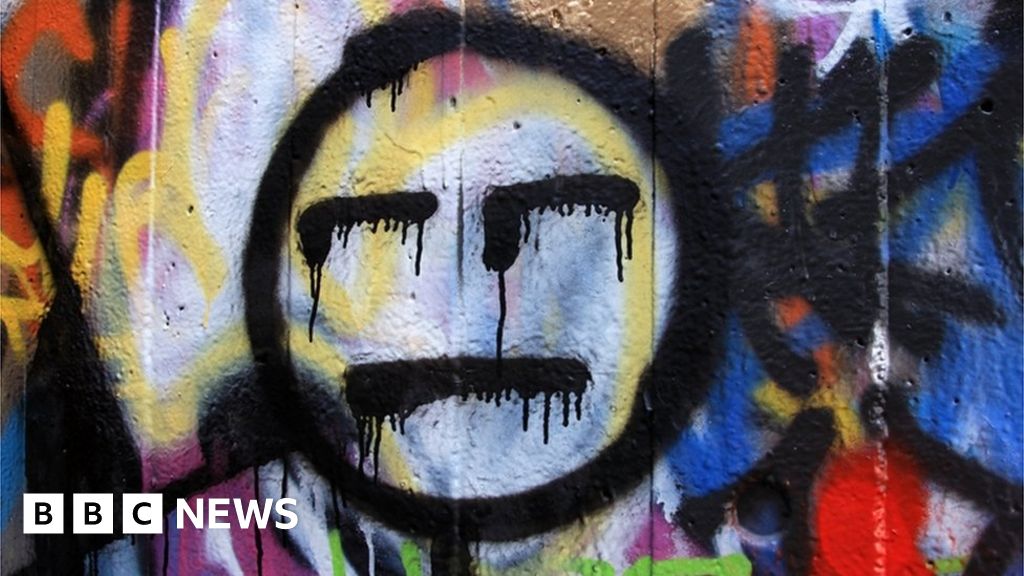The photograph captures a horizontally-oriented, graffiti-covered cement wall, characterized by visible seams running vertically. The center of the wall features a striking piece of graffiti: a black circle forming a face. This face is minimalist, with two straight horizontal lines for eyes and a straight horizontal line for a mouth, all created with black paint that appears to be dripping downwards, adding a dynamic, bleeding effect. Surrounding this central face, the wall bursts with an array of vibrant graffiti in colors like pink, yellow, red, blue, orange, white, and brown, creating a chaotic yet visually engaging background. In the lower left corner, the BBC News logo is prominently displayed, with "BBC" in white squares, each containing one of the letters, followed by "NEWS" in plain white, all-caps font.